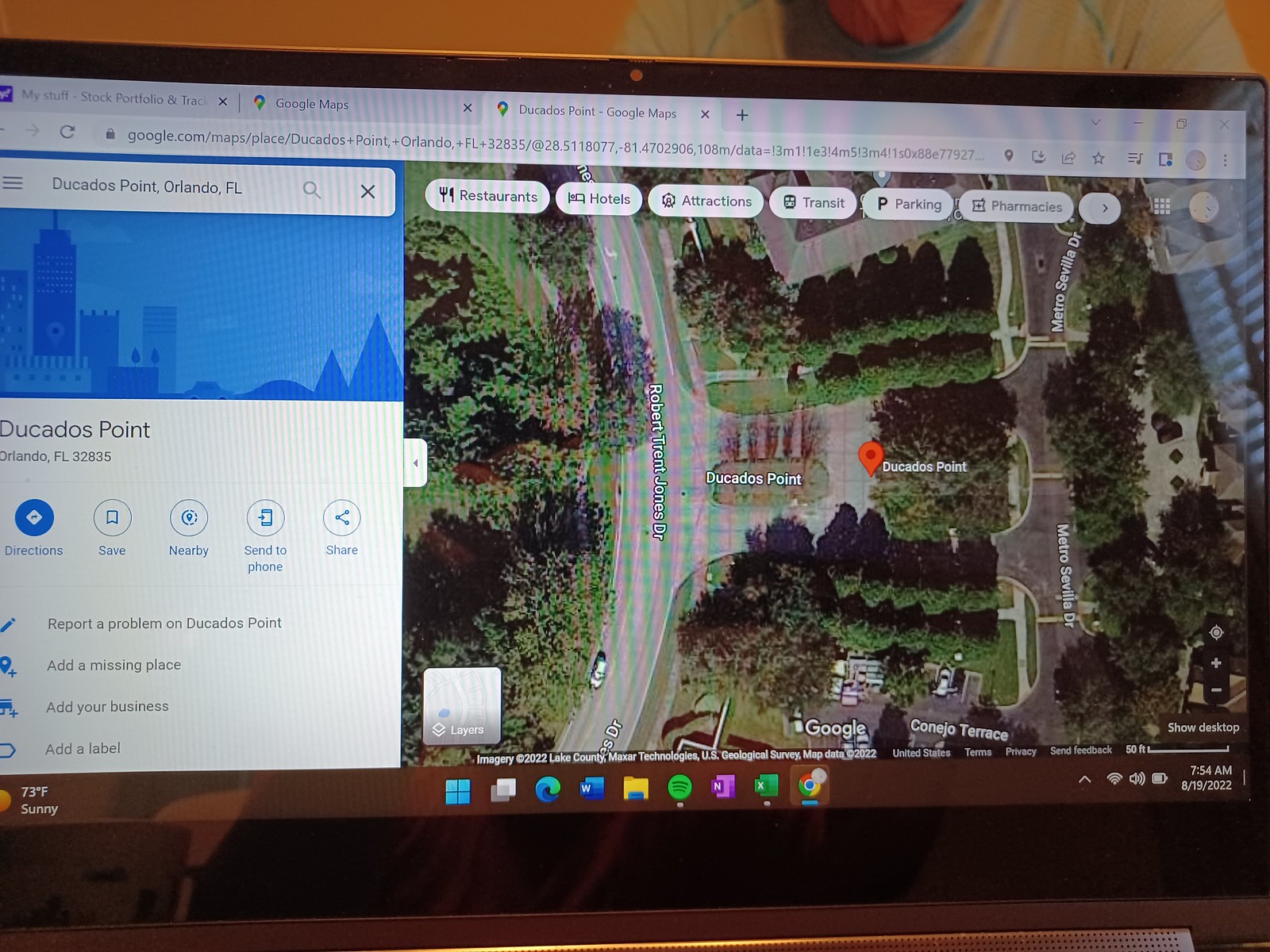This photograph captures the screen of a computer, which appears to be a desktop or a laptop based on its shape and surroundings. The primary focus on the screen is a Google Maps view, specifically of a location called Ducados Point in Orlando, Florida, with the zip code 32835. The date shown on the computer indicates the image was taken on August 19th, 2022, at 7:54 a.m. 

Prominently displayed on Google Maps are detailed street names, including a visible Robert Trent Jones Drive, with a scenic area surrounded by trees and a turnaround area. The overall map view suggests Ducados Point is a notable scenic location. Additionally, several browser tabs are open at the top of the screen, including ones labeled "My Stuff," "Stock Portfolio," and "Track," and another Google Maps tab. Details such as the black outline of the computer screen and a small section of black seen below the screen frame this focused and informative snapshot. Furthermore, in the background, the shoulders and neck of a person are visible, adding a human element to the scene.